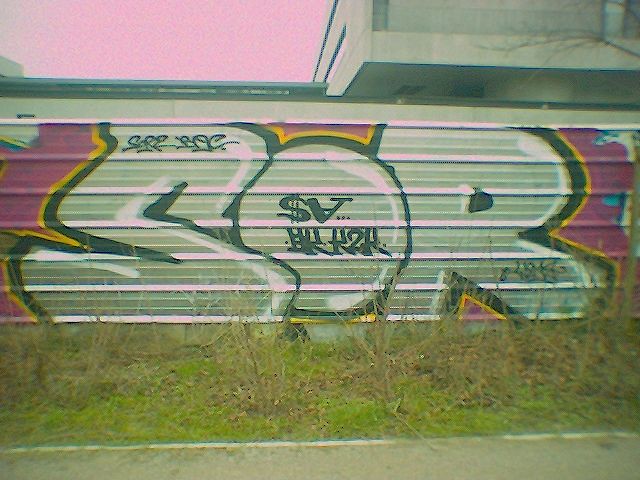This photo features a graffiti-covered wall on the side of a building, captured either early in the morning or late in the evening, as indicated by the sky's pinkish hue in the top left corner. The wall itself is predominantly gray, but the graffiti adds vibrant color: a background of magenta pink overlaid with the letters S.O.R. The letters are predominantly white or silver, accented with a black outline and a yellow border around the black. Interspersed within the 'S' are indecipherable black squiggly characters, while the 'O' contains a dollar sign, an upside-down 'A', and several other unrecognized symbols. The graffiti exhibits a light pink stripe running diagonally across the letters, adding another layer of detail.

The lower portion of the image reveals the ground, consisting of a patch of sickly, overgrown grass with brown and beige patches scattered amidst some green. The unhealthy grass is interspersed with bare, leafless bushes protruding above it. Below the vegetation, there's a segment of concrete, suggesting the presence of a walkway or road. The upper right segment of the wall transitions from the pink-painted section on the left to a plain concrete section, subtly highlighted against the early twilight or dawn sky.